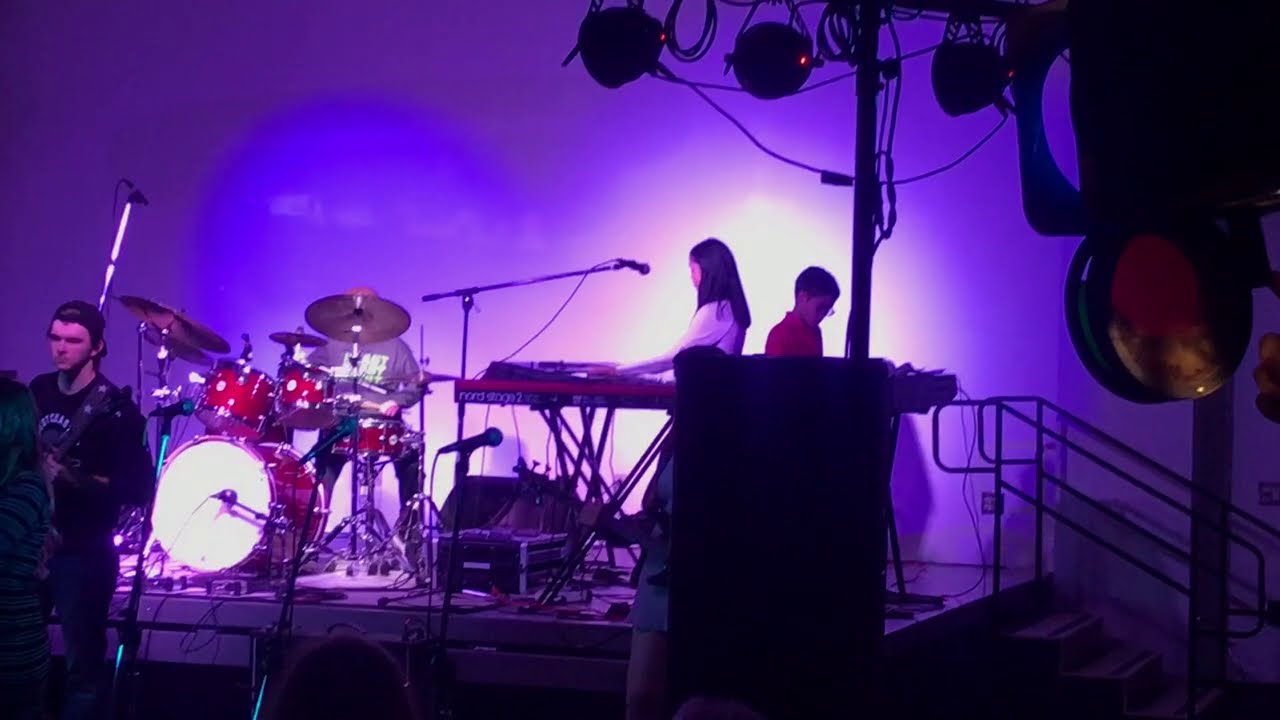The image showcases an indoor concert venue or club with a stage prominently positioned slightly off-center to the left, enveloped in a light-colored backdrop. The stage is bustling with musical instruments and performers, emphasizing a live performance setup. On the left side, a large, shiny red drum kit commands attention, with a person in a black sweatshirt playing the drums. Adjacent to the drum set, a sleek keyboard accompanied by a stand microphone stretches over it. A young Asian girl with long, straight black hair, dressed in a light-colored top, stands behind the keyboard, extending her hands toward it, poised as if ready to play or sing. To her right, a young boy wearing glasses and a red shirt stands partly obscured by a prominently placed large black speaker in the foreground. This speaker also partially conceals another individual to its left, whose left side and top of the head are barely visible. On the far left, a man with a backward ball cap, dressed in a black shirt and jeans, stands in front of the stage holding a guitar with a strap. Below the stage, the base is visible along with a small set of three stairs with a metal railing leading up to it. The whole scene is expertly lit with stage lights affixed above and to the right, casting a vibrant ambiance that suggests readiness for a concert.